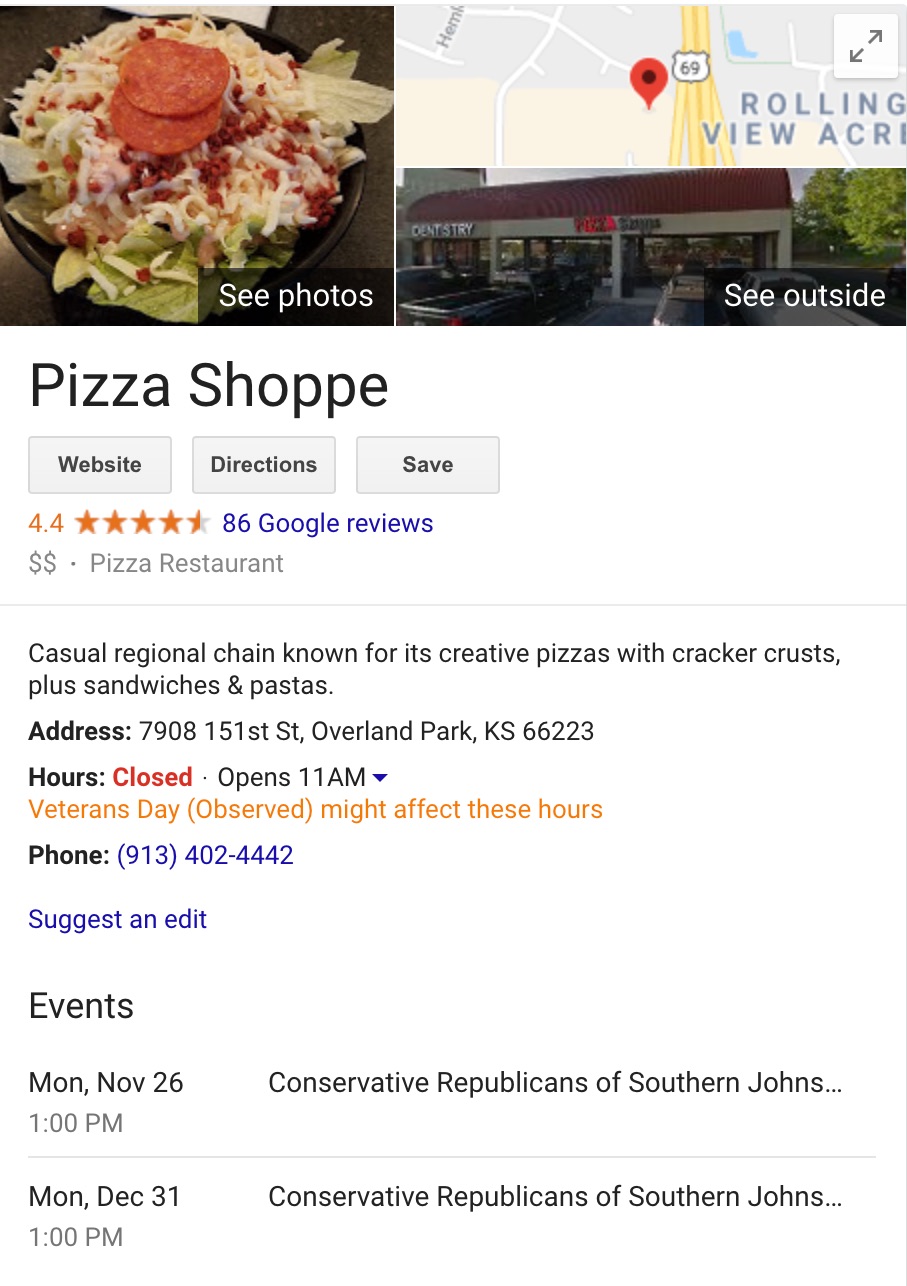This image shows a detailed search result for a pizza shop. The page is predominantly white, with various sections depicting images and information about the restaurant.

Starting from the top, there is a row of images approximately two inches from the top. One prominent image on the left side occupies about one-third of the page. It features a marble table with a black bowl filled with salad ingredients: lettuce, cheese, bacon bits, and two pepperoni slices. At the bottom right of this image, a black tab with white text reads "See photos."

To the right of this section, the upper half displays a close-up map. The map shows a red pin marking the pizza shop's location. To the right of the pin, a yellow-colored interstate runs vertically, with "Rolling View ACR" visible extending off to the right.

Below the map image is a photograph of the pizza shop itself. The building has a brown exterior with a red roof, and trees are visible on the right side. There are a few cars parked in front. Another black tab at the bottom right corner of this photo indicates "See outside" in white text.

The central portion of the page features the shop's name, "Pizza Shop," in large black letters. Below this title, three gray tabs with black text list various options: "Website," "Directions," and "Save." The shop has a rating of 4.4 stars from 86 Google reviews, highlighted in blue. Beneath this, two dollar signs indicate the price range, noted beside "Pizza Restaurant."

A thin line separates this section from the description below: "Casual regional chain known for its creative pizzas with cracker crusts, plus sandwiches and pastas."

Following this are details in bold black text: "Address" with the actual address to the right, and "Hours" with the corresponding hours beside it. An orange notice below this section warns: "Veterans Day observed might affect these hours."

Further down, contact information is provided: "Phone" followed by the number in purple. There is also a link for "Suggested edits" in purple text, and a section for "Events," listing two events with their dates, times, and names.